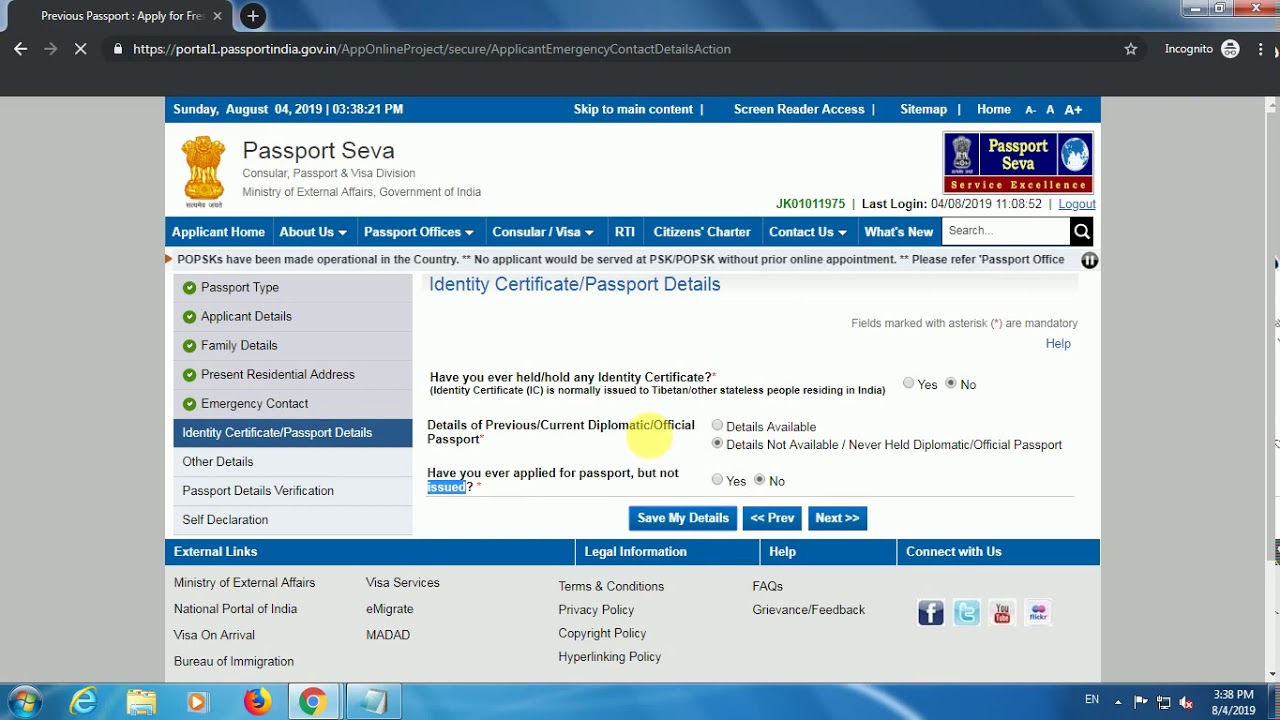The screenshot captures a browser with a single tab open, displaying the website portal1.passportindia.gov.in. The website showcases a clean design with a white background and navy blue headers featuring white text. 

At the top, the header prominently displays the time and date, Sunday, August 4, 2019, at 3:38 p.m., followed by the title "Passport Seva," part of the Consular Passport and Visa Division of the Ministry of External Affairs, Government of India. The header also includes the passport logo, depicting three golden lions standing together, and a "Passport Seva" banner located at the top right corner. 

The screenshot appears to be part of a form related to identity certificate passport details, possibly an online post or application. Users are presented with a series of questions:
1. "Have you ever held any identity certificate?" with options "Yes" and "No," where "No" is selected.
2. "Details of previous/current diplomatic official passport," with options "Details available" and "Details not available," where "Details not available" is selected.
3. "Have you ever applied for a passport but not issued?" with "Issued" highlighted in blue and options "Yes" and "No."

Below these questions, three action buttons are visible: "Save my details," "Preview," and "Next."

The bottom of the page features a footer with external links to various sections of the website, including Legal Information, Help, and Connect with Us. This section provides links to Privacy Policy, Copyright Policy, Hyperlinking Policy, Terms and Conditions, FAQs, Grievances, Feedback, National Portal of India, and Visa on Arrival. Social media links to Facebook, Twitter, YouTube, and Flickr are also present.